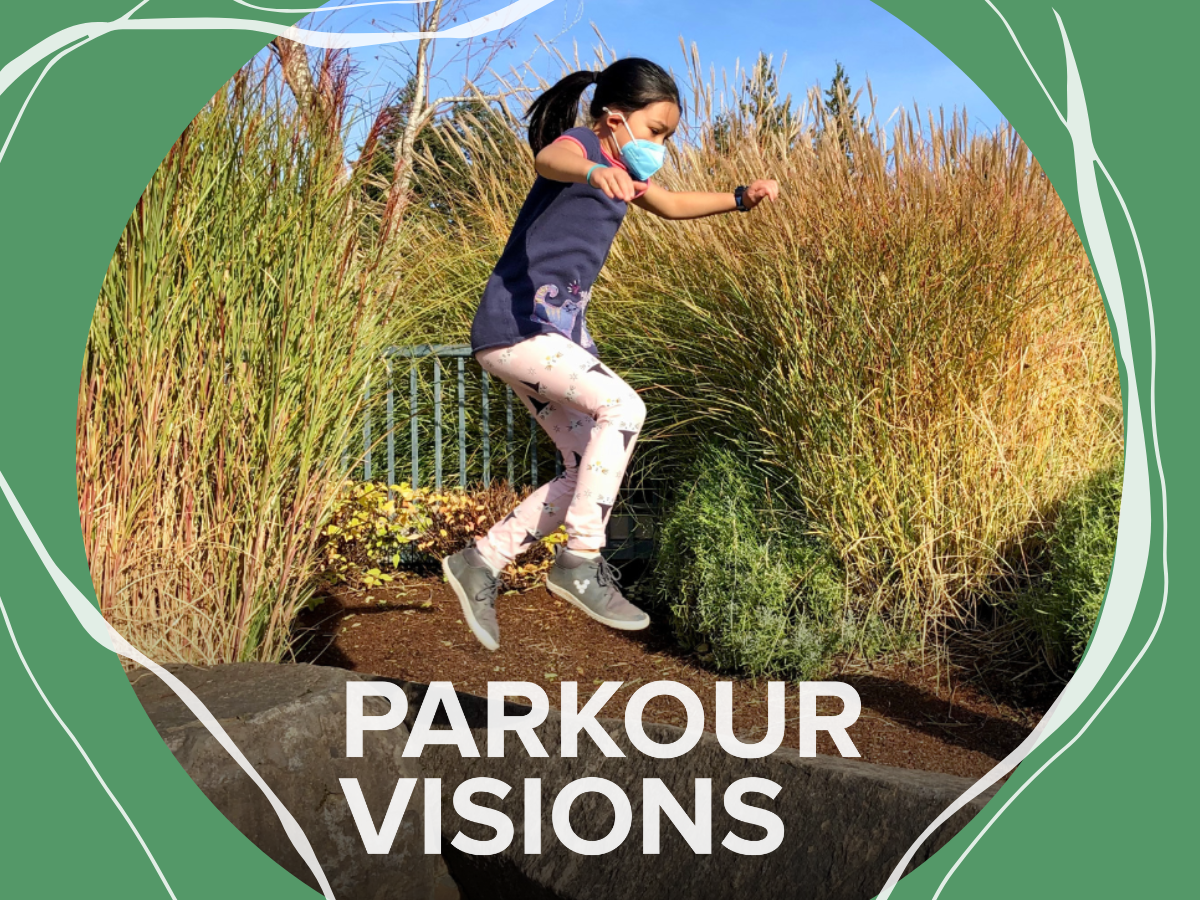The image captures a young girl mid-leap, positioned centrally. She is wearing a blue face mask and her dark long brown hair is tied up in a ponytail. She is dressed in a loose-fitting short-sleeved blue shirt and tan-colored tights adorned with designs, complemented by gray sneakers. The text "PARKOUR VISIONS" is prominently displayed in white capital letters beneath her. Surrounding her are tall, straight blades of grass in green and tan hues, with additional shrubbery and possibly a fence in the backdrop, suggesting a park setting. The scene is encased in a vertical rectangular border infused with green shades and intricate, wave-like gray lines that create a sense of movement and frame the image uniquely.